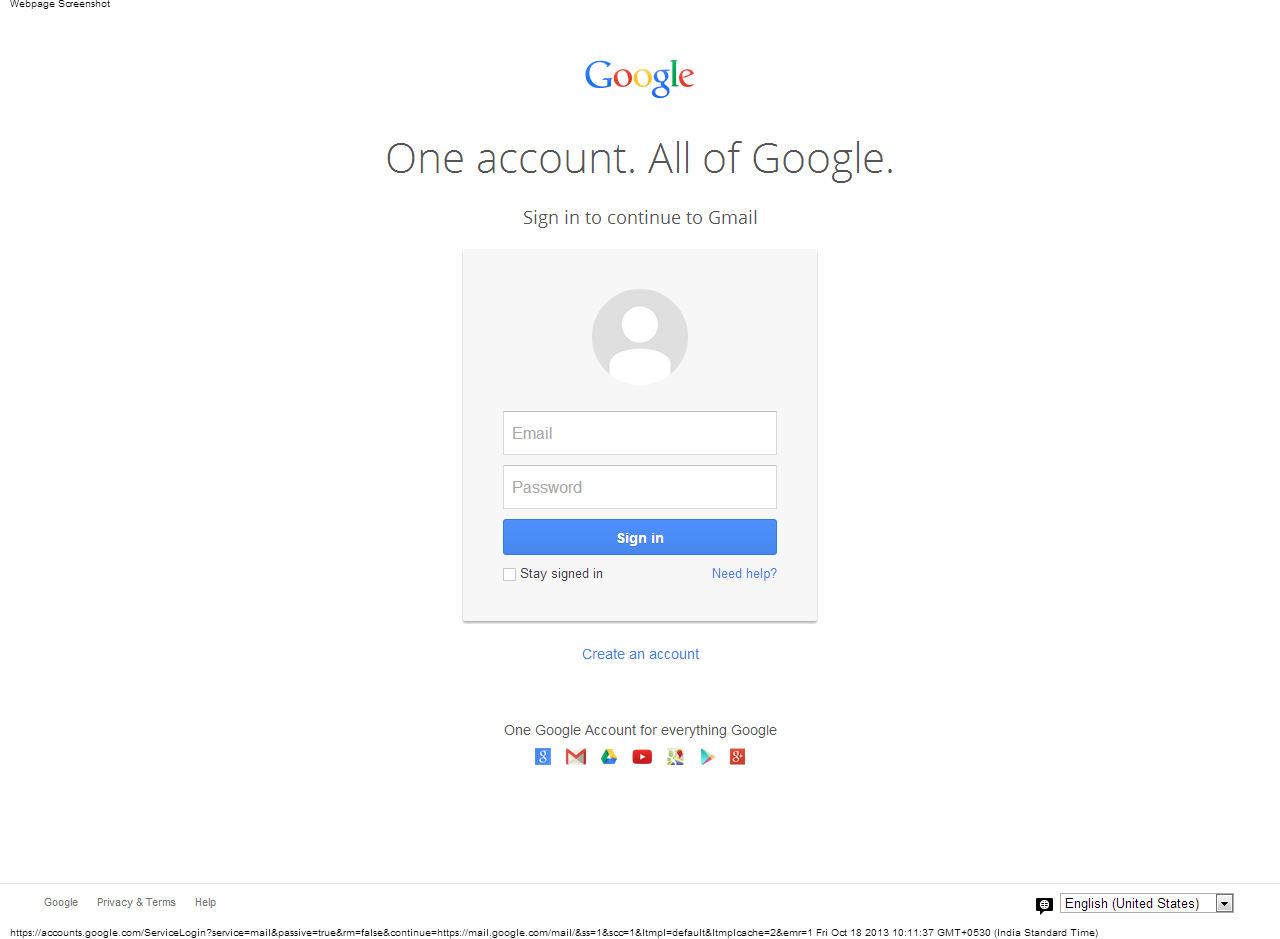The image depicts a Google sign-in webpage, featuring a minimalist design against a white background. In the upper-left corner, there is the iconic Google logo. The central portion of the page displays the bold, multi-colored "Google" text, positioned about a quarter way down from the top. Below this, in black font, is the phrase "One account. All of Google." Following this is the instruction: "Sign in to continue to Gmail."

Beneath the text, there is a light gray box with a default profile picture placeholder, depicted as a simplistic silhouette within a circular frame. Directly under the profile icon is a white input field labeled for the user's email address, followed by another white input field designed for the password. At the bottom of the form is a prominent blue button bearing the text "Sign in" in white font, inviting users to proceed with their login credentials.